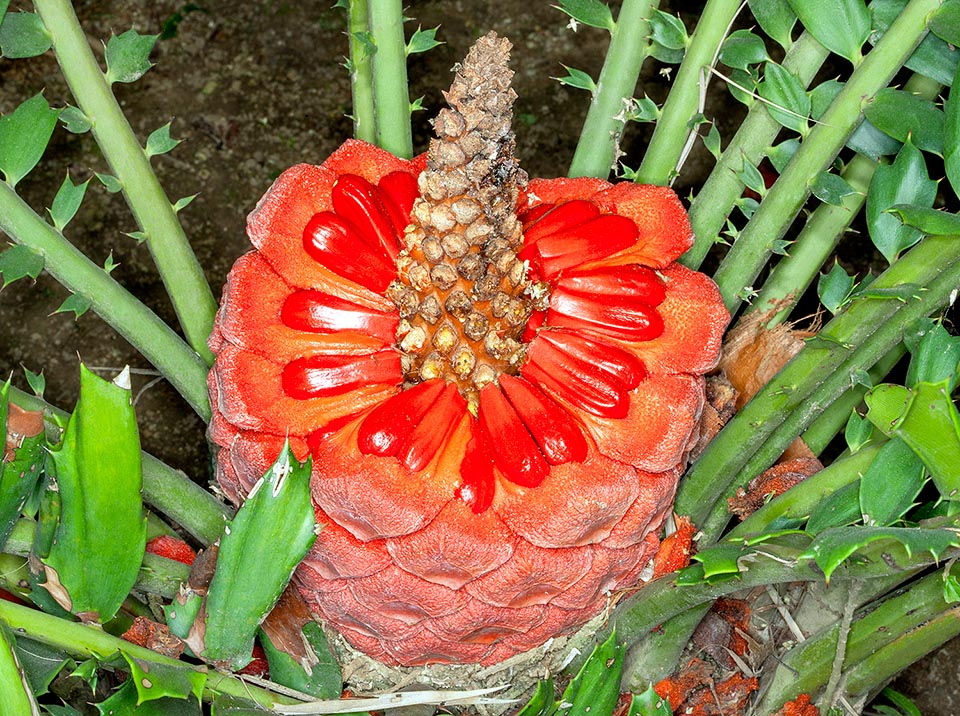In a lush garden with vibrant colors, the focal point of the image is an unusual and striking plant, likely in the early stages of blooming. Rising from a backdrop of brown soil and a network of thick, green branches, the center of the plant resembles a pineapple, but instead of the traditional yellow, it displays a spectrum of reds and oranges. The plant starts with a dusty red at the lower portion gradually blending into bright red and orange hues upwards. Emerging from its core are petal-like structures that have a layered, almost kernel-like appearance. At the very top, a pine cone-shaped cluster of budding segments unfurls, adding to its exotic look. This unique flower stands out with its pointy, vivid petals and bright green, slender leaves, creating a captivating visual spectacle.